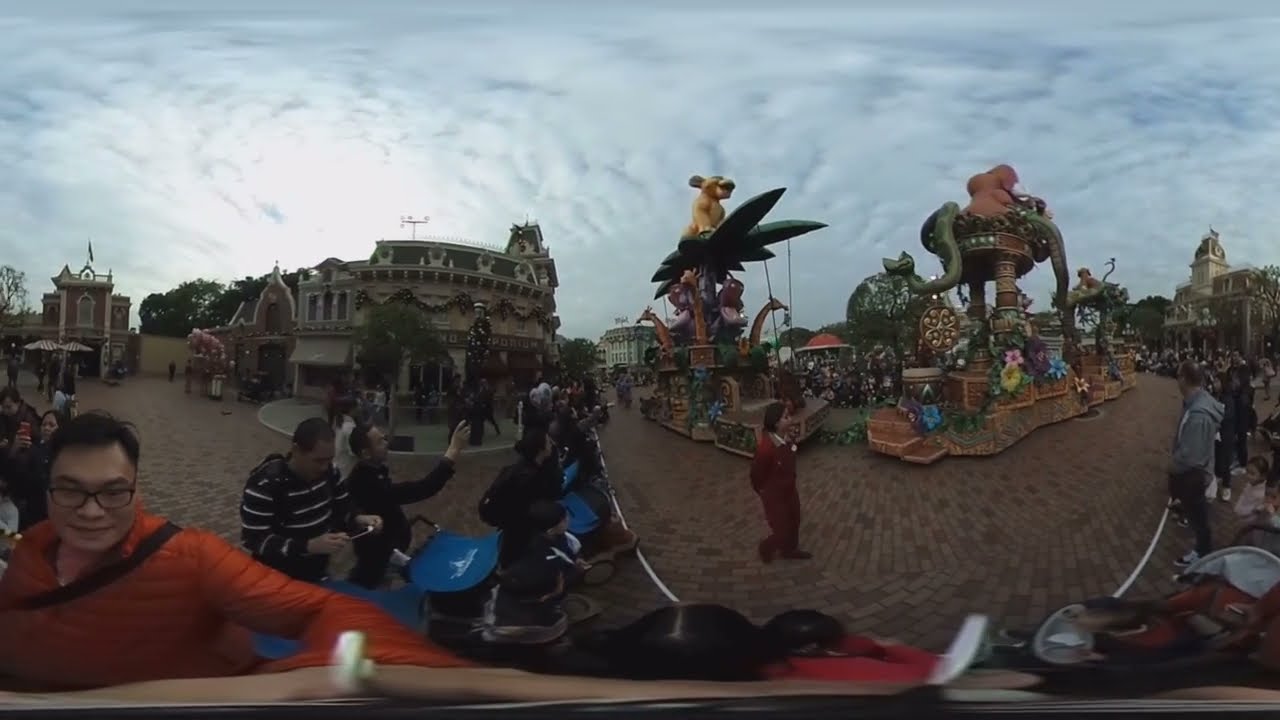The image captures a bustling Christmas parade on Main Street at Disneyland, set in a vast brick-layered courtyard. Dominating the left side of the scene is an impressively tall Christmas tree. Central to the image is a vibrant float designed to resemble a hot air balloon, adorned with gigantic artificial flowers in red, yellow, and blue. This float features a white cylindrical structure topped with a spherical element. The parade route is a loop surrounded by a dense crowd of spectators, all held back by white ropes. People dressed in various outfits, some playing musical instruments and others taking pictures, line both sides of the pathway. The background is lined with old-timey brown buildings under a cloudy sky, enhancing the festive atmosphere.